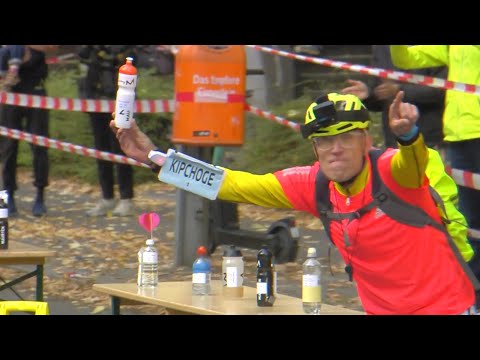In this outdoor photograph, taken in landscape orientation and possibly a screenshot from a video (evidenced by black bars on the top and bottom), the focus is on a man whose lower body is cropped out of the frame. Positioned on the right side, he is presumably a runner or cyclist, wearing a distinctive red jersey with long yellow sleeves and a matching yellow helmet that has a GoPro camera attached. He also sports clear glasses and a bright yellow backpack with visible straps. His right forearm displays a black-lettered name tag reading "Kipchoge" and he holds a white and orange water bottle in his right hand. His left hand is pointed towards the camera, suggesting interaction with it. Behind him, there's a light-colored wooden table cluttered with various water bottles in different shapes and brands. Further back, red and white striped ropes corral onlookers, affirming the outdoor race setting.